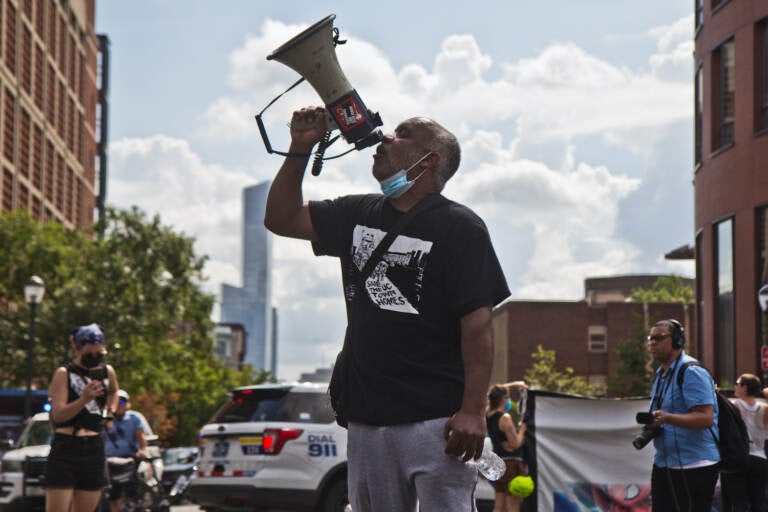In this vivid and dynamic daytime photograph, a bustling city center is the backdrop for a powerful scene of protest. The focal point is an exhausted African-American man clad in a black t-shirt with a white graphic and gray sweatpants. His bald head is tilted back, and he holds a megaphone in his right hand, raised almost vertically towards the sky, with a blue surgical mask pulled down around his chin. His left hand dangles at his side, gripping a water bottle, a testament to the day's exertion under the bright sun.

Surrounding him are fellow demonstrators, many adorned in summer attire with short sleeves and various protective face masks. Some protestors hold banners, one featuring an image resembling Spider-Man, while others are equipped with cameras and headphones, suggesting the presence of media personnel or dedicated amateur documentarians. A police SUV can be seen in the background, strategically positioned to block traffic from entering the protest area.

The scene is set against a partly cloudy sky, with light blue hues and white clouds casting soft, diffused light over the area. To the left, a sandstone building stands tall, mirrored by additional stone structures and a towering skyscraper in the background. Adding a touch of nature amidst the urban landscape, a dark green leafy tree is visible along the street, contrasting with the man-made surroundings. This image captures the essence of a hot day in the city, filled with passionate voices and a collective call for change.